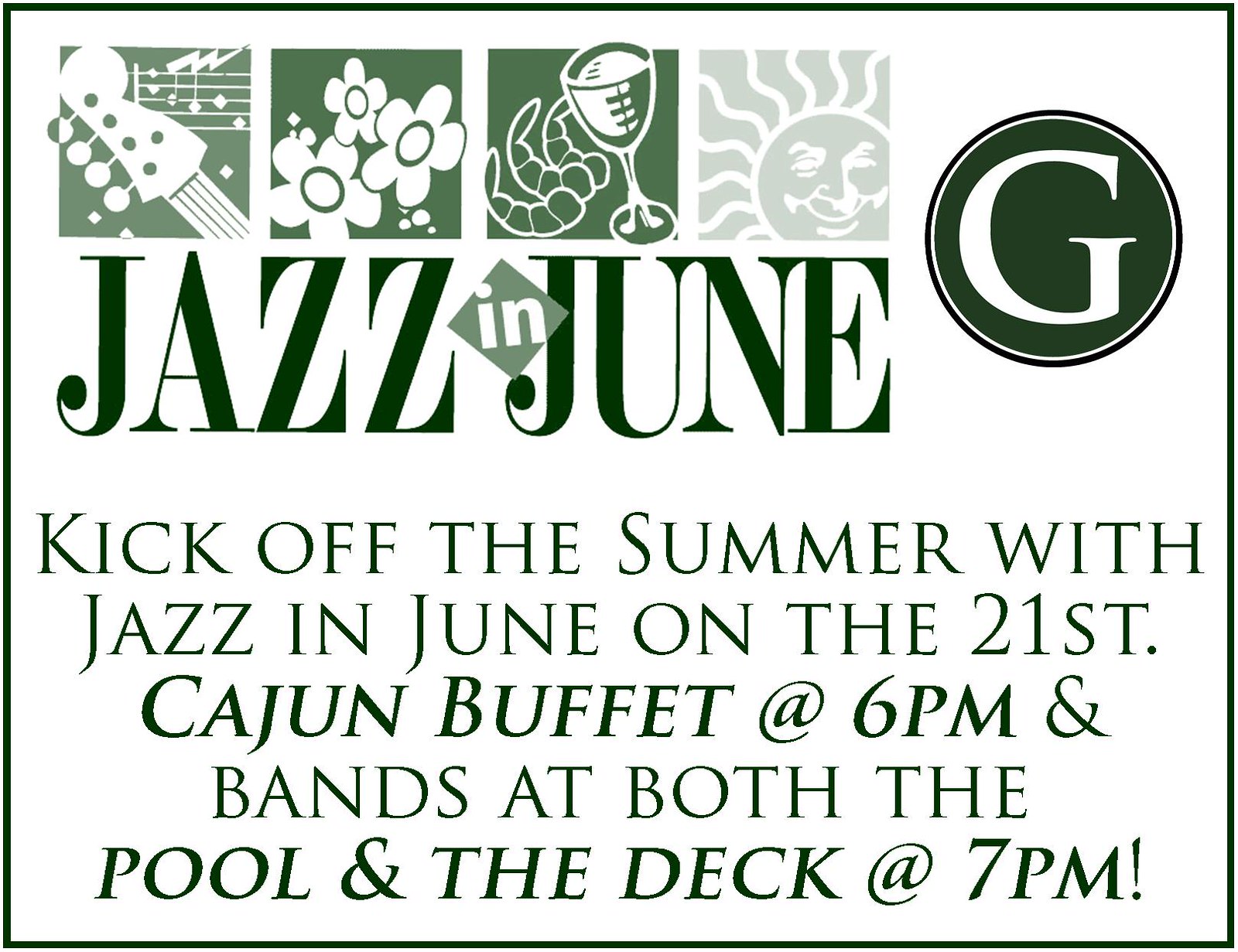This advertisement for an event is outlined in dark green with a white background. The top left features four small images in squares: a guitar, flowers, shrimp in what appears to be wine, and a sun, resembling clip art. Adjacent to these images is a green circle encompassing a white letter "G." Below this visual arrangement, the caption reads "Jazz in June" in bold. Further down, in thinner green font, the text invites attendees to "kick off the summer with Jazz in June on the 21st," highlighting a Cajun buffet at 6 p.m. and live bands performing at both the pool and the deck at 7 p.m. The location or city for the event is not specified in the image.